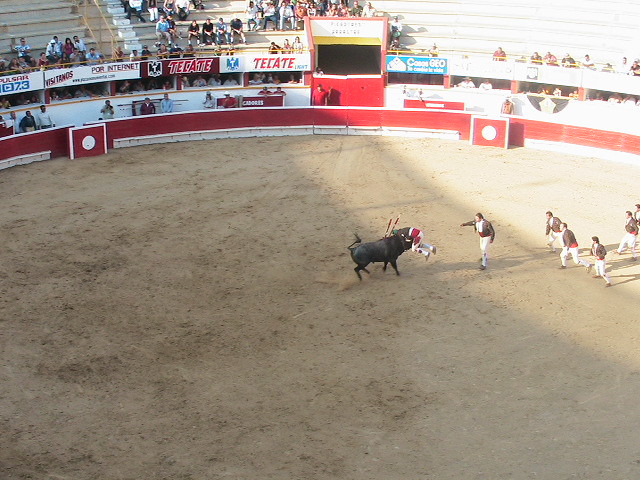This photo captures a dramatic moment during a bullfight in a sparsely populated Spanish stadium. Shot from above, it offers a clear view of the brown dirt arena enclosed by a red wall. At the center of the scene, a black bull is shown lifting a matador whose groin is precariously positioned over the bull's face. The matador is clad in a gray jacket, white pants, and a red sash, appearing distressed but uninjured. Nearby, another matador points towards the bull, while three more in typical attire rush forward, with two additional men approaching from the side. The upper portion of the image shows a curved red concrete barrier separating the arena from the spectators, who sit sparsely in gray concrete seats beyond a white arch. Signs, including one that reads "Tecate," decorate the stands, adding context to this intense and dynamic spectacle.